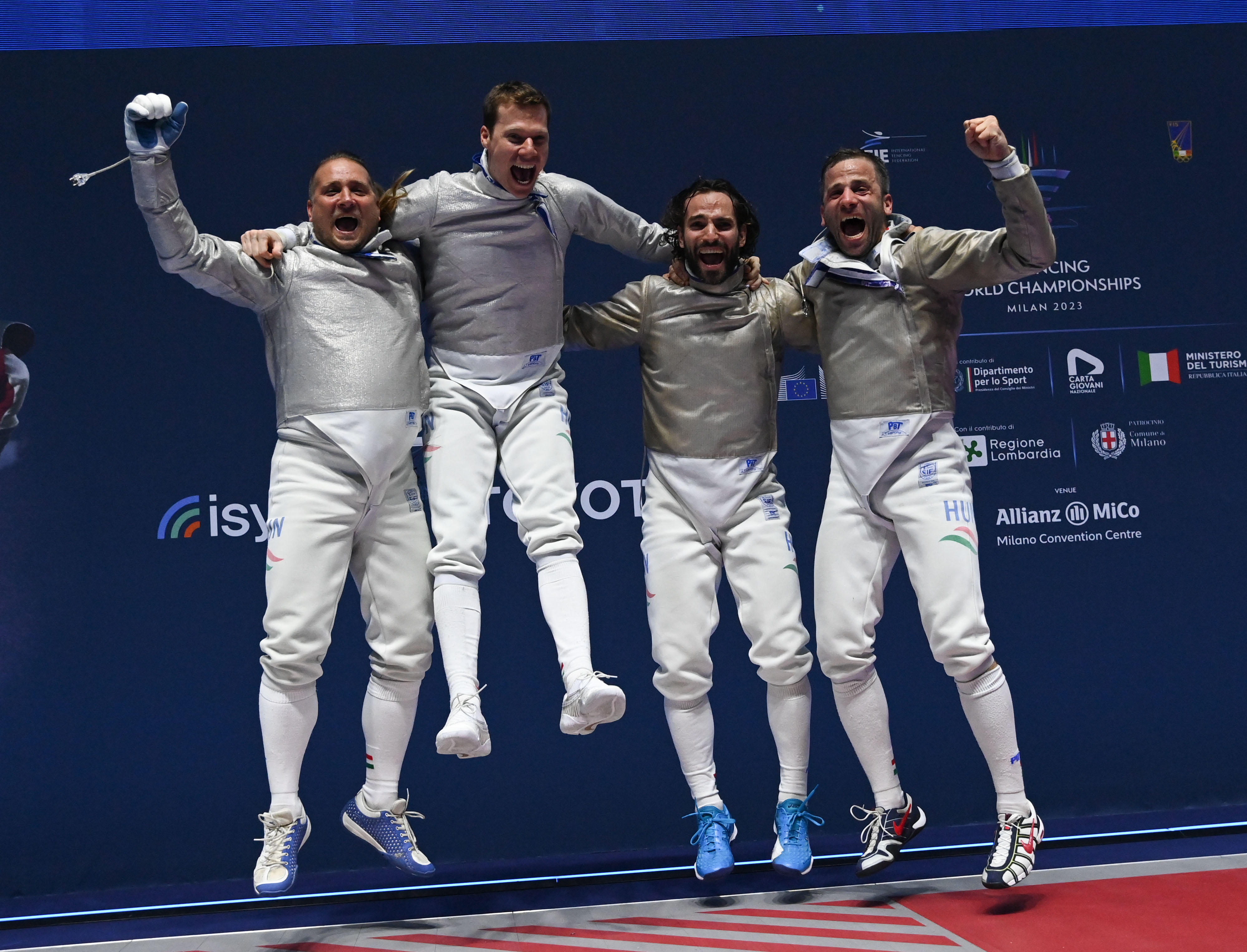In the image, four men are captured mid-jump, celebrating joyfully with their mouths wide open and fists raised. They are all dressed in silver metallic shirts and white pants, typically worn in fencing, along with colorful sneakers—two pairs blue, one mostly white, and one white with black and red accents. The second man from the left jumps notably higher than the others, showcasing their exuberance. The men are closely adjoined, some holding each other, and two have their fists up. The one on the left wears a single glove. The backdrop is a blue wall adorned with various advertisements, partially obscured but recognizable as promoting the World Championships in Milan 2023, including a visible 'Toyota' logo. The ground beneath them features a red and white striped pattern.